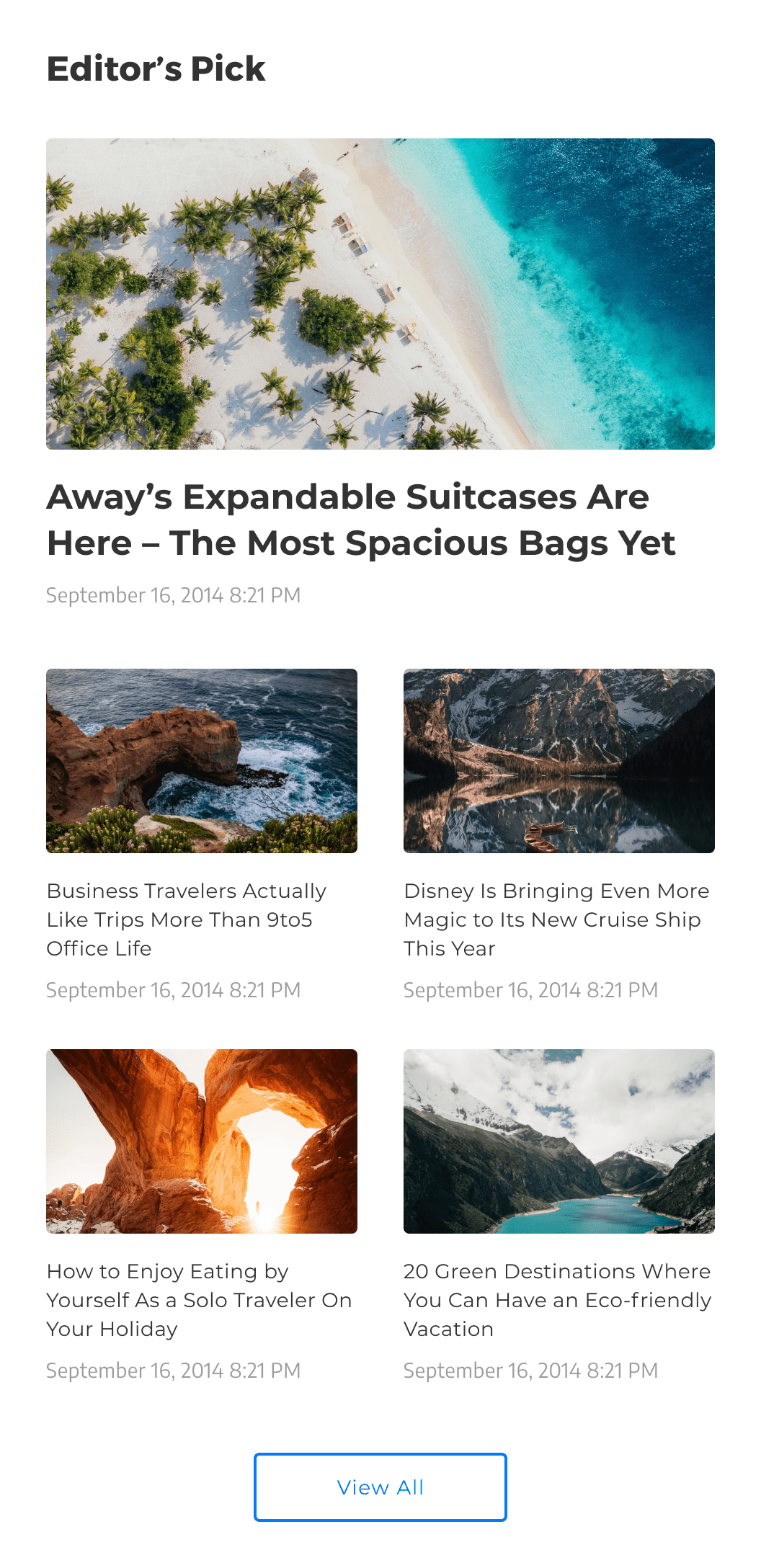The image features a header labeled "Editor's Pick" at the top. Below the header is a captivating photograph of crystal-clear blue water along a serene beach adorned with palm trees. Prominently displayed is a title announcing, "Away's Expandable Suitcases Are Here - The Most Spacious Bags Yet," marked with a timestamp of September 16, 2014, at 8:21 PM. The image is surrounded by four additional article headlines, each with accompanying pictures and the same publication time and date.

1. The first headline reads, "Business Travelers Actually Like Trips More Than 9-5 Office Life." This is paired with an image of a picturesque ocean scene with intriguing rock formations.
2. The second headline, "Disney Is Bringing Even More Magic to Its New Cruise Ship This Year," is set against a stunning mountain landscape background.
3. The third article, "How to Enjoy Eating by Yourself as a Solo Traveler on Your Holiday," features a breathtaking view of giant rock formations creating a natural arch.
4. The final headline, "20 Green Destinations Where You Can Have an Eco-Friendly Vacation," showcases a tranquil body of water encircled by majestic mountain ranges.

A clickable button labeled "View All" is situated at the bottom, inviting readers to explore further.